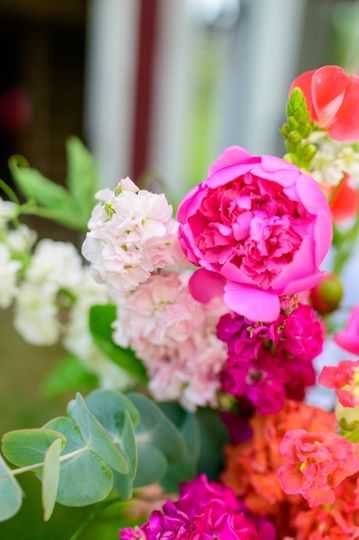This close-up portrait captures a vibrant, mixed bouquet of flowers. The central bloom, likely a pink peony, is surrounded by a variety of other flowers that may include carnations and geraniums, displaying a rich palette of pink, peach, coral, orange, purple, and white hues. The lower portion of the image shows green leaves, possibly from eucalyptus, situated towards the bottom left. The flower arrangement fans out from the center towards the bottom right. The background is a soft blur of green, red, and white tones, seamlessly blending into each other, leaving the setting indistinct. The image, likely taken in a garden or a flower shop, focuses solely on the exquisite details of the flower petals, making the precise location unidentifiable. The absence of any text ensures that the viewer's attention remains on the colorful, detailed floral composition.